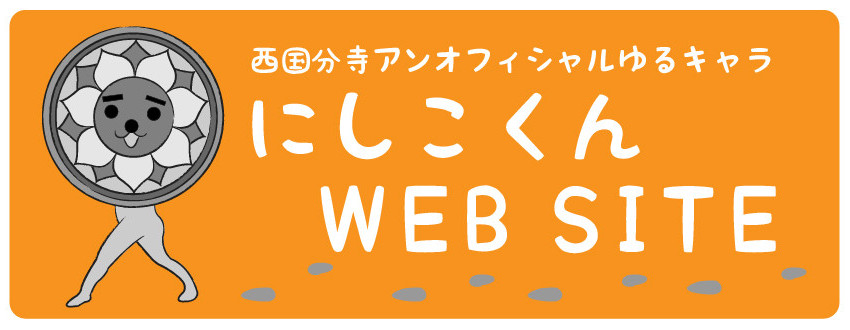This image features a horizontally oriented advertisement or business card with a dominant orange background. On the left side of the image, there is an intricate graphic design. The central element of this design is a large gray and white outlined circle containing a cheerful dog face with black eyes, a round nose, and a gray tongue sticking out, giving it a sun-like appearance with floral petals radiating outward. Below this circular face is a pair of gray legs, resembling a figure walking. These legs appear dog-like and contribute to the playful nature of the graphic. 

To the right of this circle, there are several rows of white text. The first two rows contain Chinese characters or some other type of Asian script. Below this, in larger white text, the word "website" is displayed prominently. At the very bottom of the graphic, extending from right to left, are small blue footprints, indicating the path of the walking figure. This element gives the design a dynamic, continuous movement across the sign.